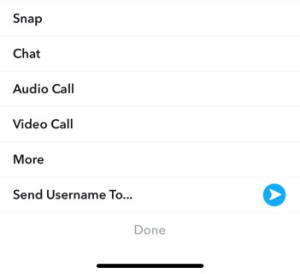The image depicts a user interface on a plain white background, showcasing various communication options arranged vertically along the left side. From top to bottom, the options include: "Snap," "Chat," "Audio Call," "Video Call," "More," and "Send Username to...". Each option is separated by a subtle, faint horizontal line that extends from left to right across the interface, providing clear divisions between choices. 

The layout ensures that each option is flush to the left, with ample spacing, making it easy to distinguish and read each one. Notably, the "Send Username to..." option is followed by an ellipsis ("..."). 

The only splash of color in the user interface is a small, white arrow enclosed in a blue circle located next to the options, signifying a selectable button. Centered at the bottom of the interface, there is a "Done" button in a muted gray color, underneath which is a thick black line that does not span the entire width of the interface but is centered, extending slightly before and after the "Done" button.